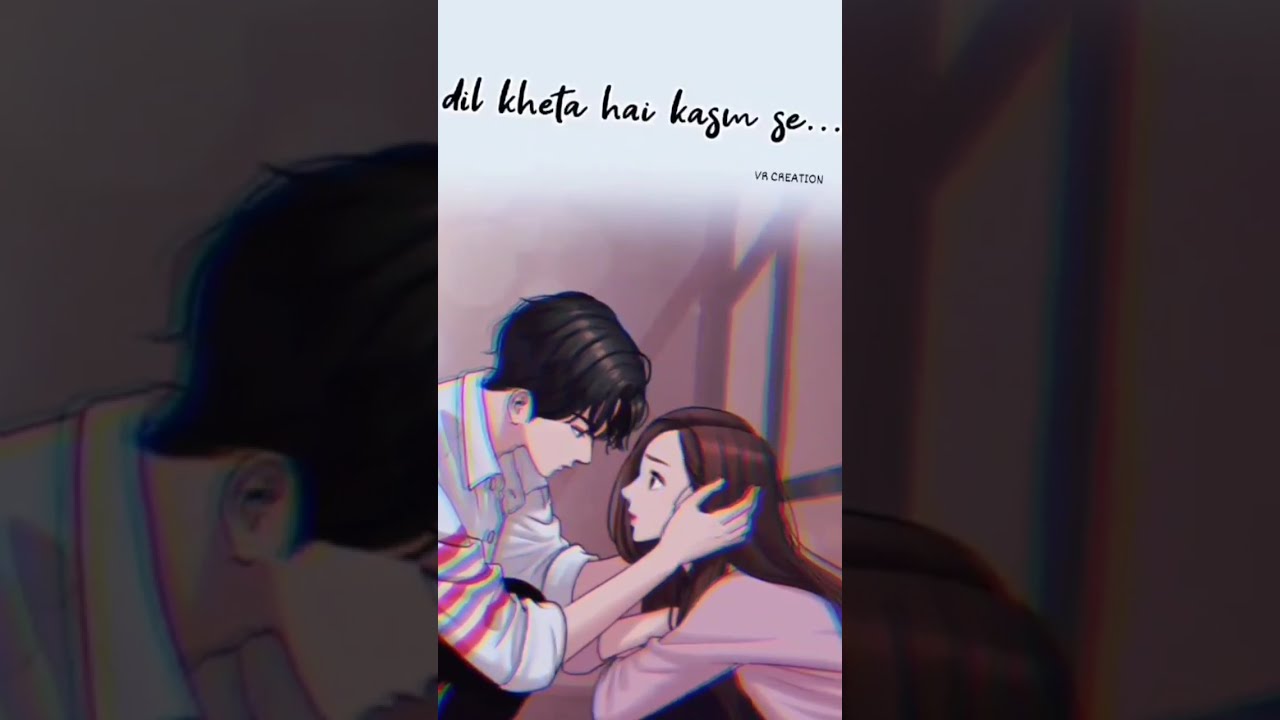The image depicts a highly detailed, vertical anime scene that appears to be part of a digital cell phone display. The central image features a young boy and girl in an emotional interaction. The boy, with strikingly dark black hair that falls over his eyelids, is kneeling and wearing a white collared polo shirt with dark pink and purple stripes on the short sleeves, which are rolled up to his elbows. He has light skin and a worried expression as he gently holds the face of the young girl. The girl, with long, dark brownish-reddish hair parted in the center, is sitting cross-legged, looking up at the boy with a similarly concerned look on her face. She has fair skin and is wearing a pink shirt. The background of their interaction is a purplish-pink hue with faint, square-like grid shadows.

Above the scene, in bold black letters on a light gray band that stretches across the width of the image, is foreign text that reads "D-I-L K-H-E-T-A H-A-I K-A-S-E-N S-E..." Below this line, in smaller text, it appears to say "V-R Creation." The entire image is framed between two enlarged, darker copies of the same scene, with the left side showing the back of the boy's head and the right side showing the top of the girl's head. The background suggests a foggy, outdoor environment, adding to the dramatic and intense mood of the scene. The dimensions of the image are roughly six inches wide and three inches tall, separated into three distinct sections that contribute to its manga or comic book aesthetic.